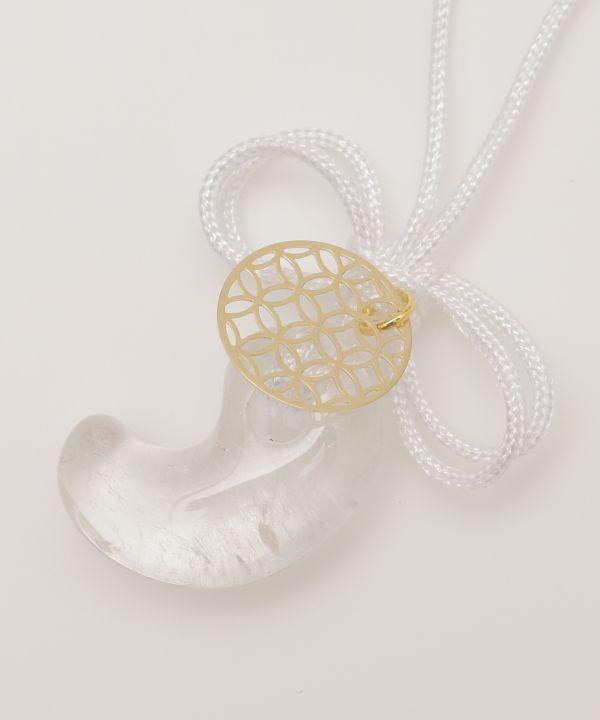The image features a delicate, thin white rope with a textured, silky appearance. This rope has been meticulously tied into two elegant bows. Two strands of the rope extend upwards, disappearing out of the frame at the top right corner. Resting on top of the bows is a piece of intricate jewelry, resembling a round, gold-toned earring adorned with loops and triangular shapes crafted from the metal. This ornament is attached to the rope with a matching gold clasp, giving it the illusion of being part of the necklace. Positioned underneath the piece of jewelry is a small, white, peanut-shaped object with a textured surface, adding a unique and whimsical element to the composition.